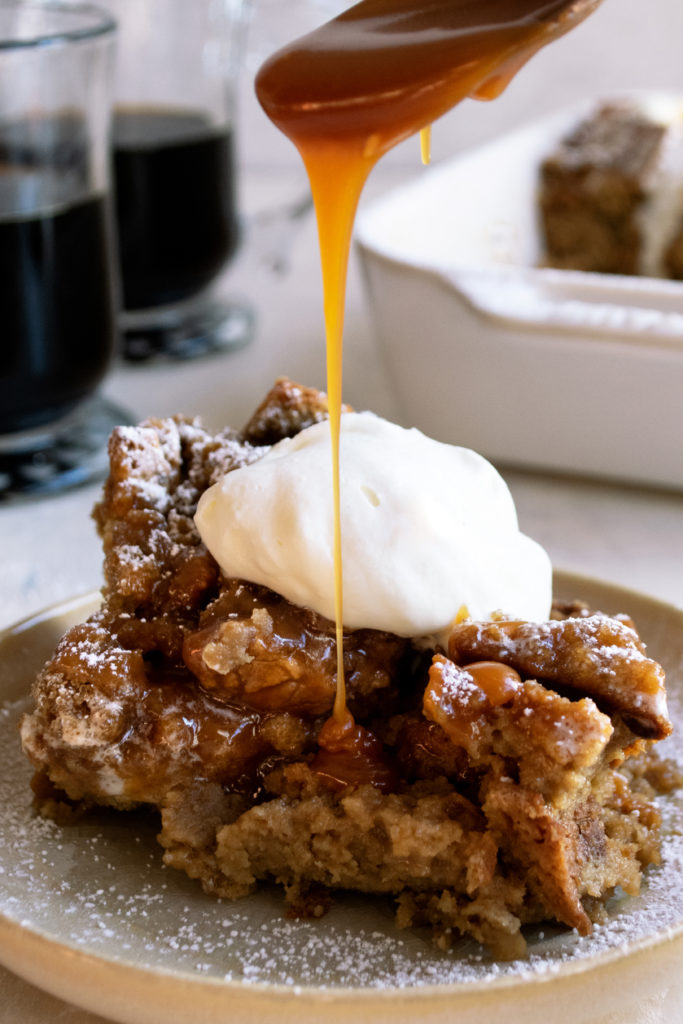This close-up color photograph captures an irresistible dessert, potentially a caramel apple crumble or gingerbread cake, sitting on a beige ceramic plate. The dessert is brown, crumbly, and has a slightly sticky texture, adorned with a generous dollop of whipped cream on top. Sprinkled powdered sugar adds a delicate touch to both the dessert and the plate. A stream of melted caramel is caught mid-drizzle from an unseen container, cascading over the dessert from top to bottom. In the background, two clear coffee mugs filled with dark liquid and a white dish with more dessert are visible on a white table surface.